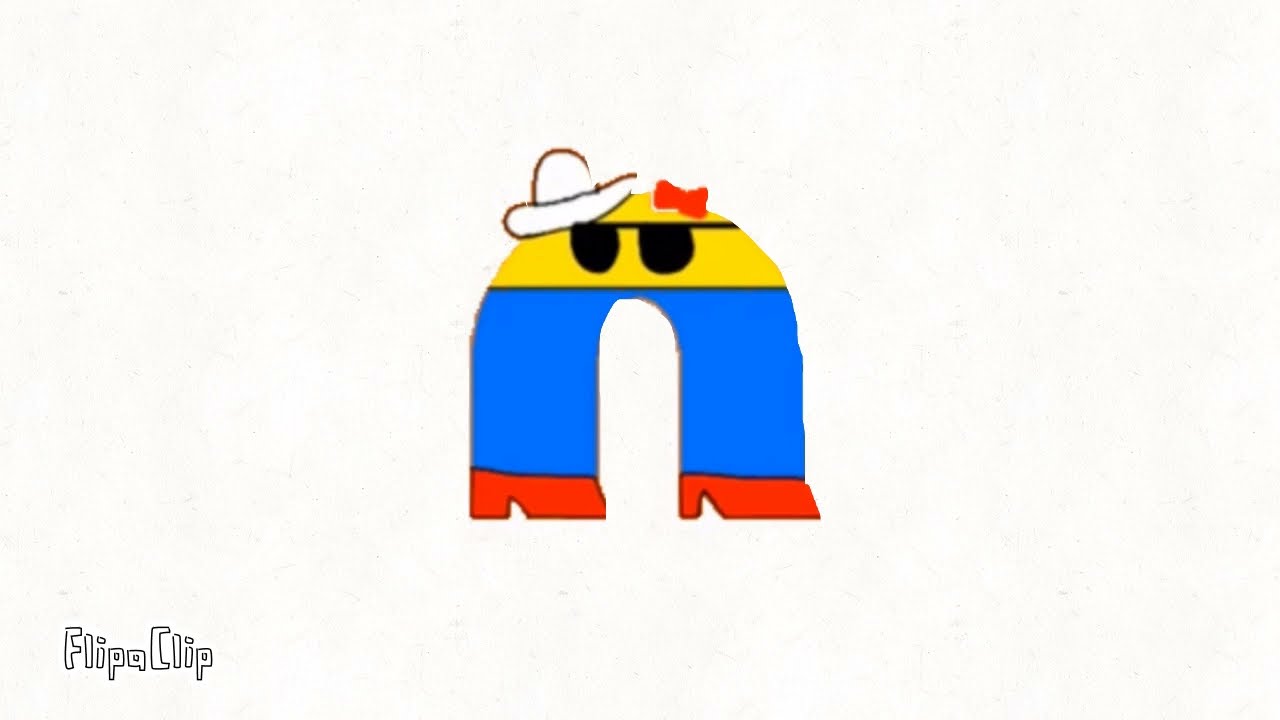The image is a wide rectangular digital artwork set against an off-white background. At the center, it features an upside-down U-shaped figure resembling a person. The top of the U forms the head, which is yellow and adorned with black sunglasses, a red bow, and a white cowboy hat on the right side. The curved part of the U represents the torso, covered in a red shirt. The lower parts of the U resemble legs dressed in blue jeans, ending in red high heels that point to the right. In the bottom left corner, outlined in handwritten black font, are the words "FLIPACLIP."